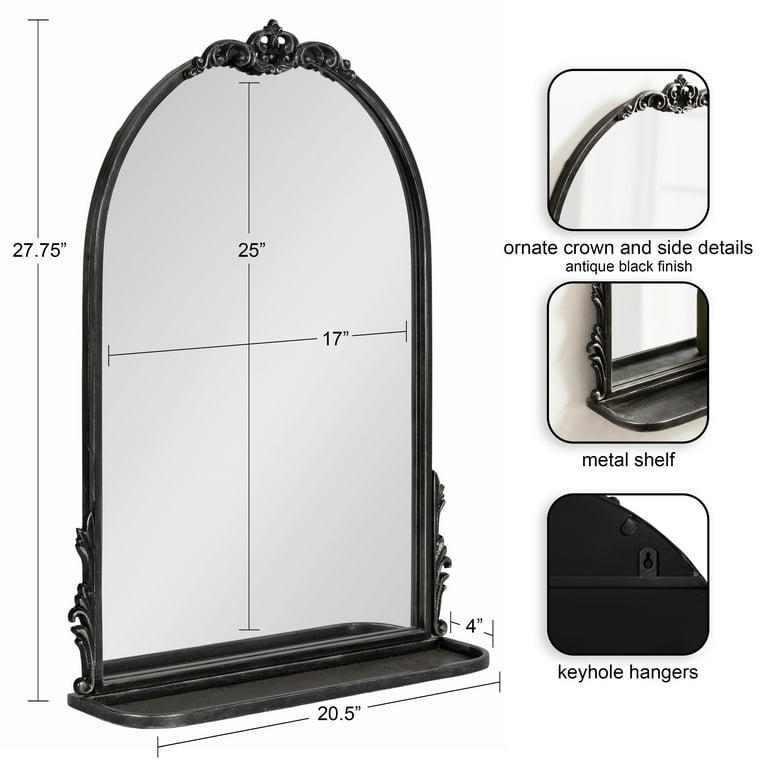In this detailed black-and-white image of an ornate mirror, prominently positioned on the left side of the frame, we observe a mirror with an antique black finish. The mirror features a black frame and base, and is divided into four distinct parts, each showcasing different dimensions and decorative details. The top of the mirror is rounded, crowned with an ornate design, while the bottom part includes a small, integrated metal shelf. Measured from top to bottom, the external length of the mirror is 27.75 inches, with the internal glass length being 25 inches. The width of the mirror from edge to edge is 20.5 inches, while the internal breadth of the reflective surface is 17 inches. Overall, the mirror is 4 inches thick. Additional features highlighted include keyhole hangers for mounting, positioned likely at the back, and detailed side embellishments that enhance its antique aesthetic.